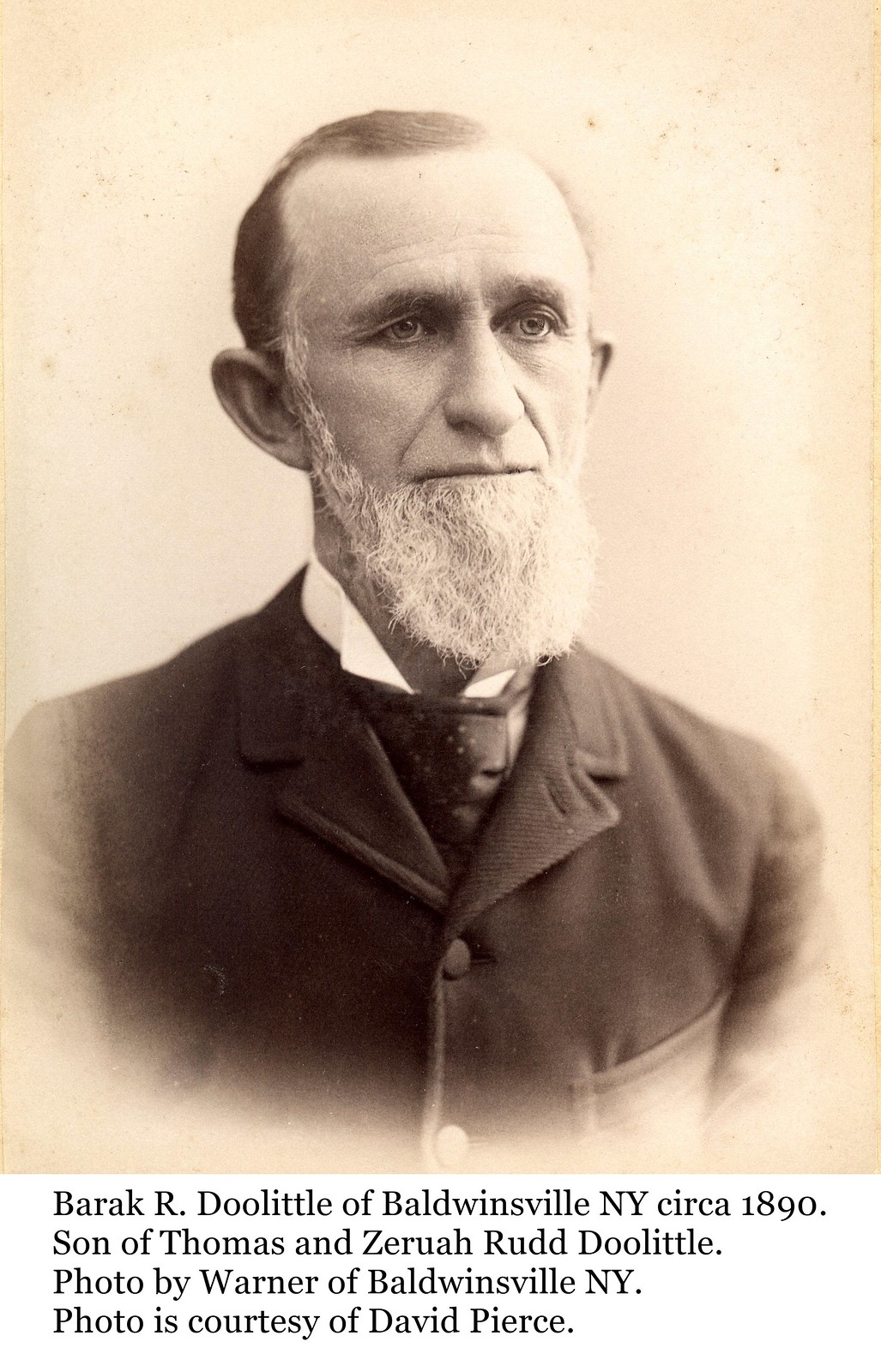This is an old, faded black and white photograph of an older man with a white beard, large ears, and thinning, dark hair on top and on the sides, featuring prominent sideburns. He is wearing a thick, dark overcoat with buttons and a pocket, along with a white shirt and a visible tie underneath. The photograph is aged, showing stains and spots, and has a gradient background that ranges from peach to light tan, becoming lighter at the bottom, where parts of the subject's arms appear faded. The man's expression is somber as he gazes directly into the camera with dark eyes. Below the image, text reads: "Barack R. Doolittle of Baldwinsville, New York circa 1890, son of Thomas and Zeruiah Rude Doolittle. Photo by Warner of Baldwinsville, New York. Photo courtesy of David Pierce."